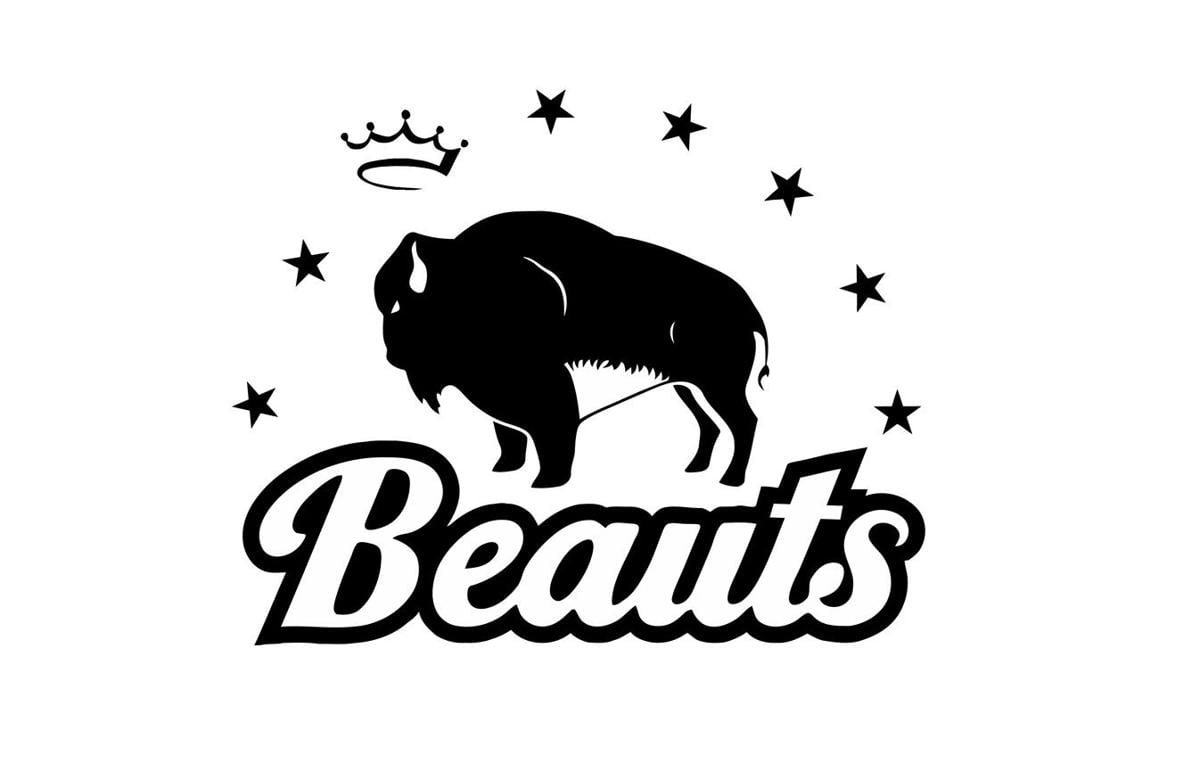The image features a logo set against a white background. Central to the design is the black silhouette of a robust bull, oriented to face left. The bull is distinguished by stark white accents - its horns, eyes, and belly stand out against its dark body. Above the bull, seven black stars form an arch; two stars appear on the left, then a crown, and five more stars continue the arch to the right. Beneath the bull, in elegant cursive white letters outlined in black, is the word "Beauts" with a capital 'B'.